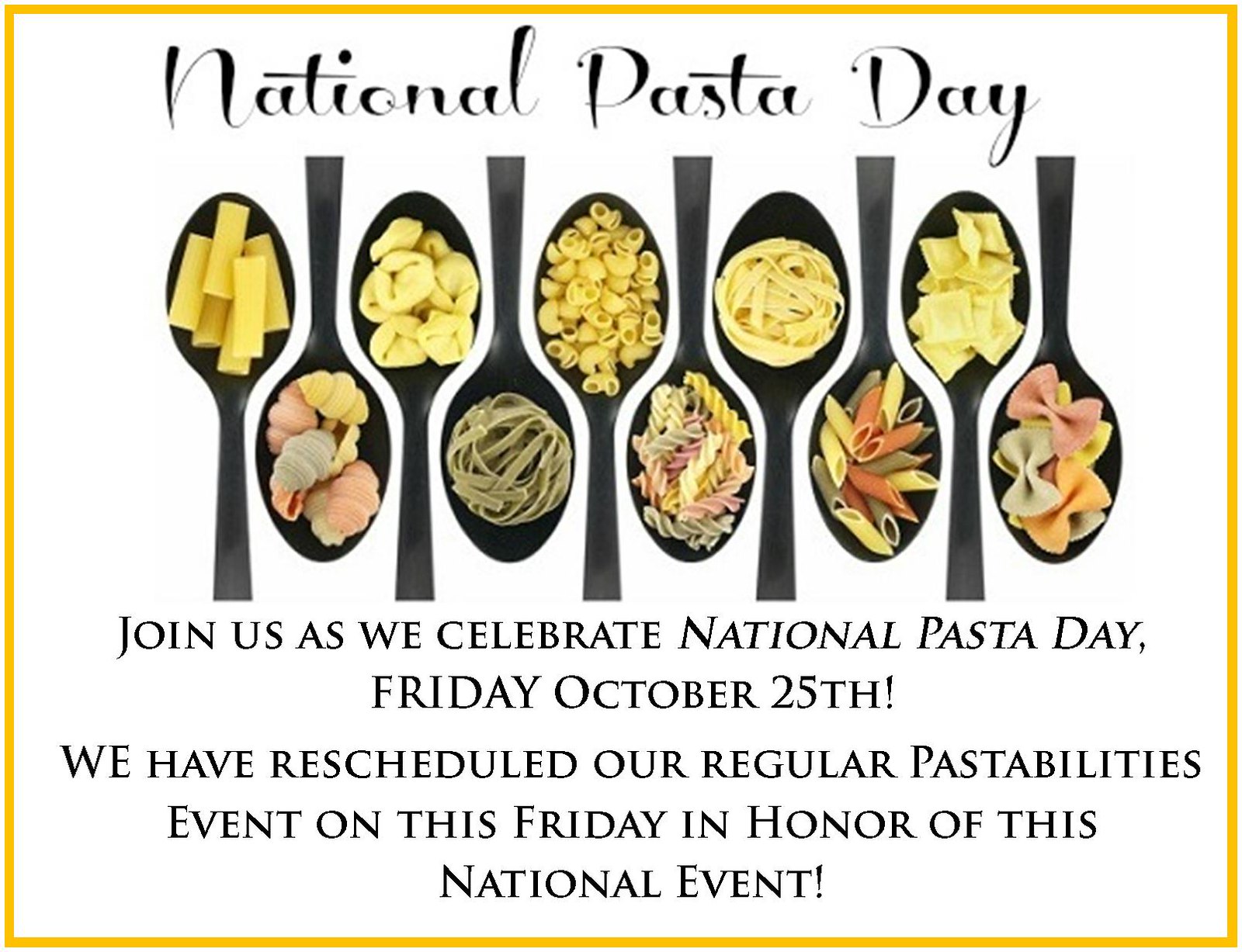The image is an advertisement for National Pasta Day, framed by a thin gold line. Titled "National Pasta Day" in black letters at the top, it features 10 black spoons placed side by side in the center, alternating in direction. Each spoon showcases a different type of pasta, with varieties including long tubes of rigatoni, shell-like penne, dumpling-shaped pasta, green fettuccine, and a butterfly or bowtie shape in mixed colors of red, green, and pink. Below the spoons, it invites viewers to join the celebration on Friday, October 25th, and notes that regular Pastabilities events have been rescheduled for this national event.